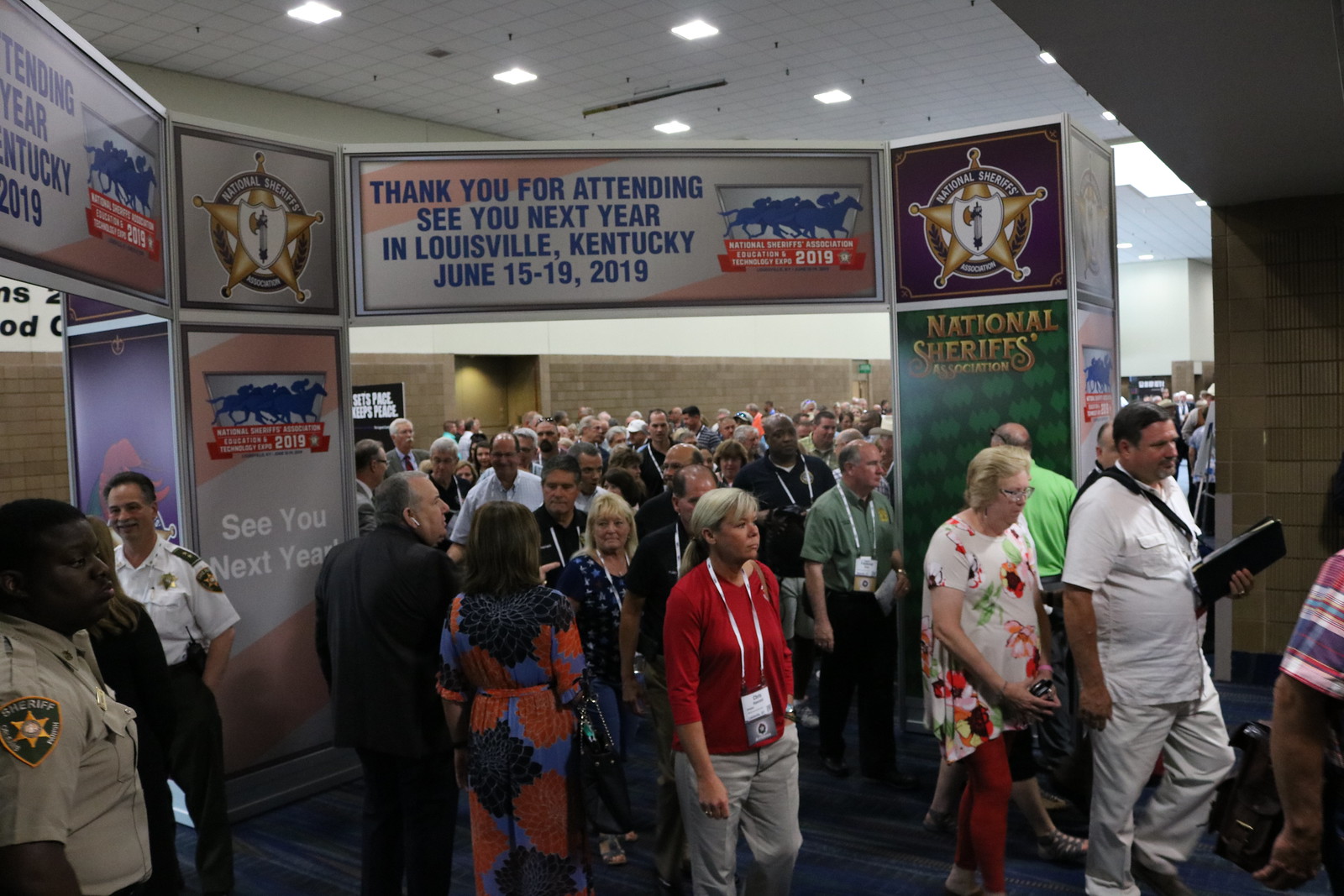This image captures the bustling exit of a National Sheriff's Association convention, likely the culmination of the event, as emphasized by the crowd of about a hundred people. It appears to have been taken inside a building and features a large archway adorned with various signs. The prominent central sign, with a white and red background and blue text, reads "Thank you for attending, see you next year in Louisville, Kentucky, June 15th to 19th, 2019." Beneath this central text, a red banner states "National Sheriffs Association Education and Technology Expo 2019," flanked by gold five-pointed sheriff stars and logos featuring a badge with a hatchet emblem.

The scene is vibrant and colorful, with the crowd dressed in a mix of attire showcasing a spectrum of colors including brown, orange, black, red, white, pink, and blue. Among the crowd, a man holding a folder and individuals wearing passes can be observed, contributing to the casual and informal atmosphere of the snapshot, which seems to have been taken by an onlooker. Additionally, a uniformed sheriff's officer wearing a khaki shirt is visible in the bottom left corner, further emphasizing the official nature of the event. The overall scene exudes the energy and camaraderie of a well-attended convention coming to a close.